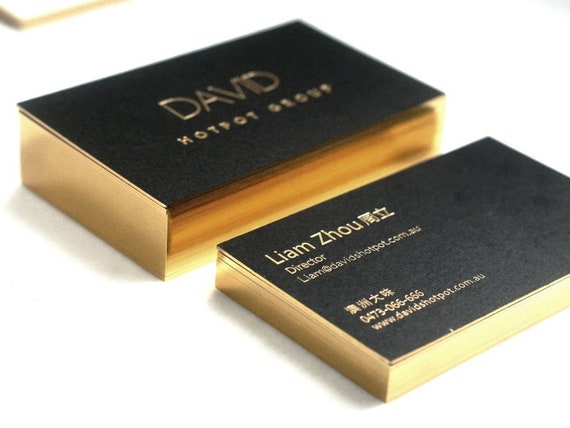This photograph captures an elegant stack of high-quality business cards belonging to Liam Xu, Director at DavidsHotPot.com.au. The cards are made from black paper and feature gold debossed text, giving them a luxurious and professional appearance. The card prominently displays "David Hot Pot Group" in gold script on one side. On the other side, visible from a secondary, shorter stack, it includes Liam's name, title, email (Liam@DavidsHotPot.com.au), phone number (04730666666), and the website (www.DavidsHotPot.com.au). Additionally, there are some Mandarin characters. The edges of the cards are also gilded in metallic gold, seamlessly blending with the gold script and making the entire design cohesive and highly reflective.